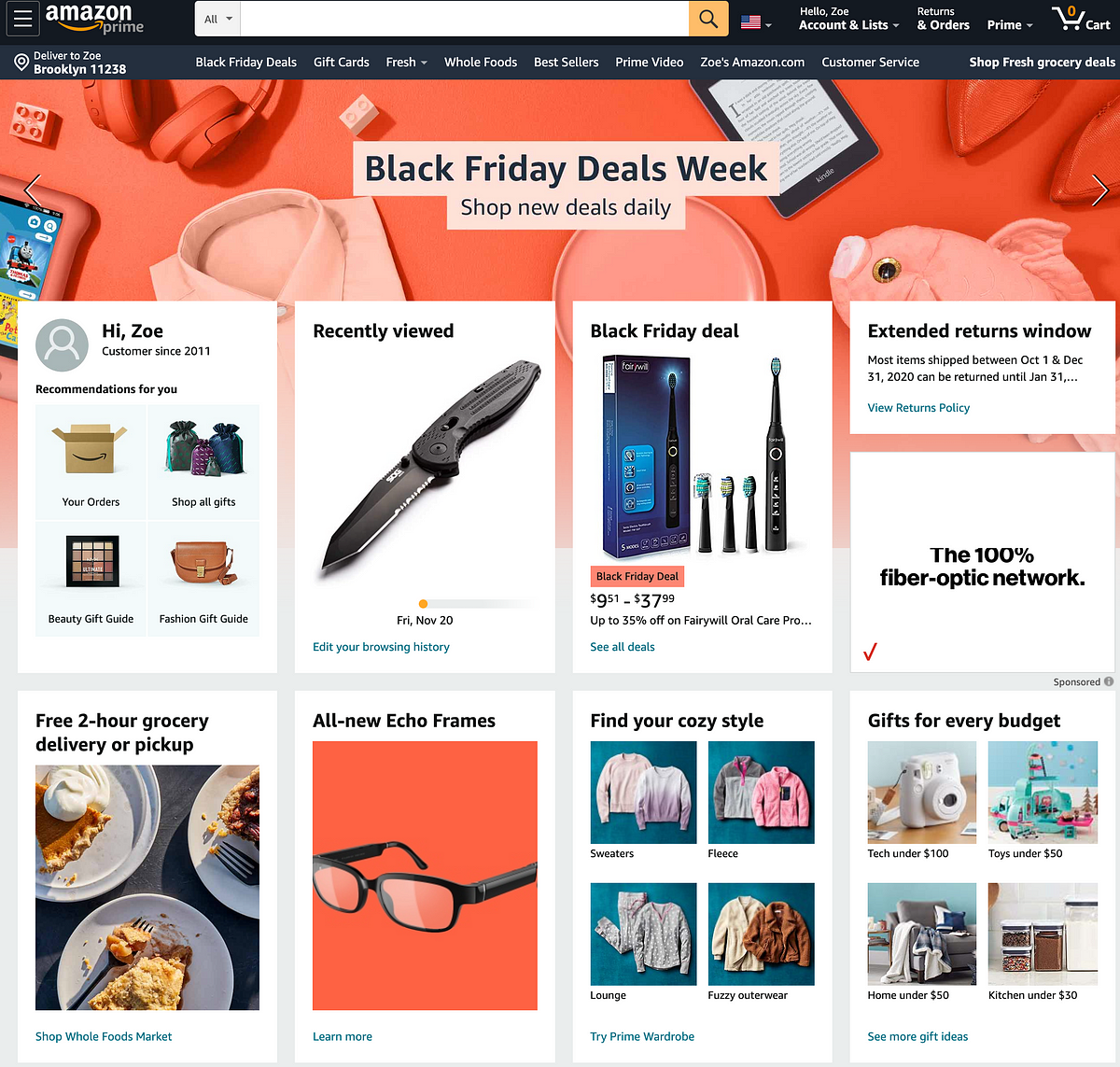The top left corner features the Amazon logo in white with "Prime" below it, accompanied by the signature small orange arrow. To the right, a large search bar is prominently displayed, followed by the small image of the United States flag. Next to these elements are links for Accounts & Lists, Orders, Prime, and a cart icon showing a count of zero items in orange.

Below this header, a banner announces "Black Friday Deals Week" with the tagline "Shop new deals daily." The background of this section is predominantly red, highlighting a pair of red headphones, a pink shirt, a pink fish toy, and an Amazon Kindle.

The next section features a white background and a personalized greeting: "Hi, Zoe, customer since 2011. Recommendations for you." Adjacent to this is a box titled "Recently Viewed," showcasing an image of a black knife.

Further along, another box highlights a "Black Friday Deal" for an electric toothbrush. 

In the bottom row, a promotion for "Free two-hour grocery delivery or pickup" features images of various pies, including a slice of pumpkin pie topped with whipped cream. Next, the "All-new Echo Frames" are showcased within a red box, displaying sleek black frames.

Following this, the "Find Your Cozy Style" section is adorned with images of cozy sweaters. The final box, "Gifts for Every Budget," features a variety of items such as cameras, toys, and a chair adorned with throw blankets.